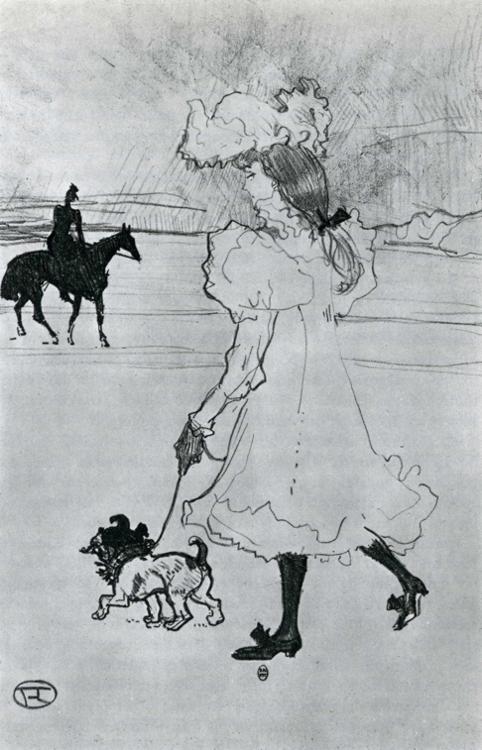The image is a black and white pencil drawing of a woman walking. The woman is slightly off-center to the right, donning a long, white frilly dress with puffy shoulders that extends beyond her knees. She wears black hose and black shoes adorned with bows. Her long hair cascades down her back, tied with a bow, and she sports a frilly hat. Her face is visible from a three-quarter profile view, showing one eye. In her hand, she holds a leash attached to a small dog with a black head, gray collar, white body, and black tail. The background features a silhouette of a person riding a horse, with sketch-like hills and straight lines. There appears to be the artist’s signature in the lower left corner of the image, adding a final touch to this simple yet detailed composition that evokes a 1700s-1800s impressionistic style.